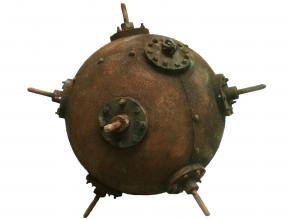The image showcases a rusted, spherical sea mine positioned on a pristine white background, implying it is not submerged but placed on dry land. The mine's surface is weathered and bears a reddish-brown hue, suggestive of extensive rust. It features six prominent, evenly distributed metal spikes protruding from various angles: one pointing up, one to the right, one downward, and one towards the viewer, along with two others symmetrically placed. Rivets delineate the mine, arranged along the seams where the segments are joined and around the bases of the spikes. One particular circular section on the mine appears designed to attach a chain, indicating it could be anchored and floated in water. The detailed craftsmanship is evident in the alignment of the rivets and the precise placement of the spikes, making the image a detailed study of this antique maritime weapon.